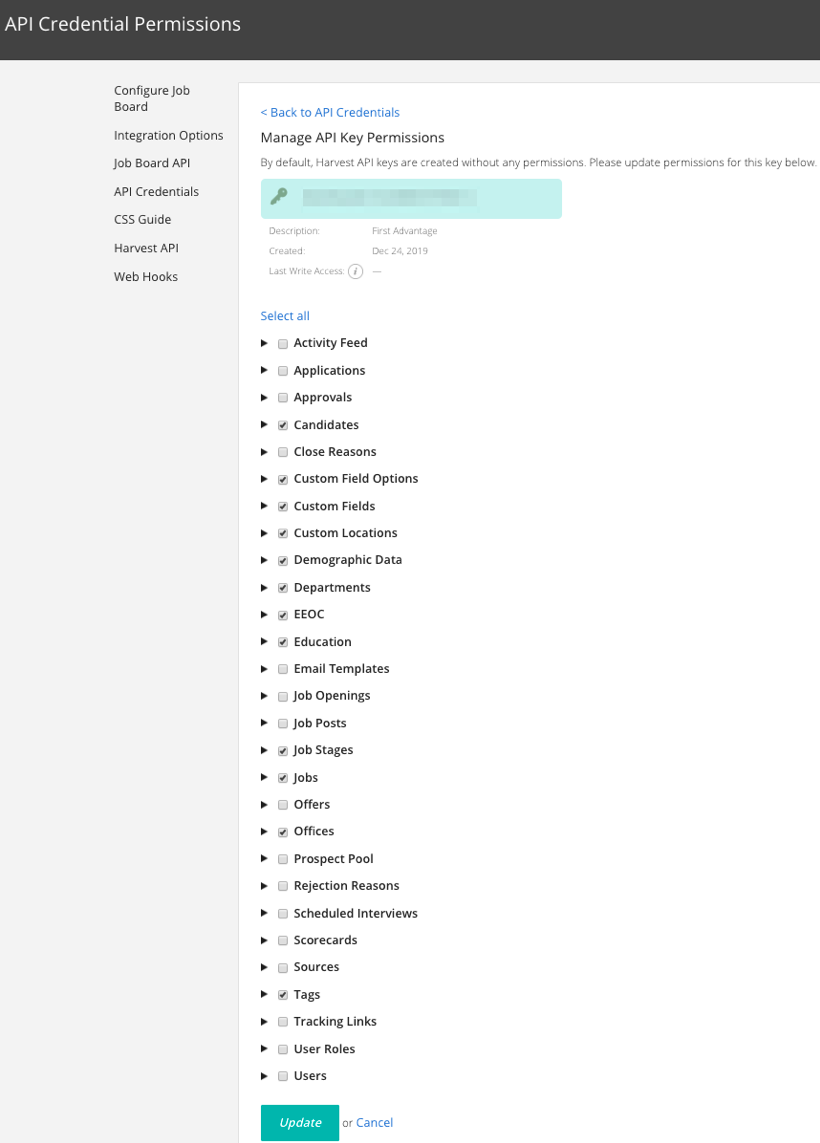The image is a smartphone screenshot displaying a website's API credential permissions page. At the top of the screenshot, there is a black banner with white text. On the left side, there is a tannish-colored section, and underneath it, navigation tabs are arranged vertically. These tabs include "Configure Job Board," "Integration Options," "Job Board API," "API Credentials," "CSS Guide," "Harvest API," and "Webhooks."

The right side of the image features a white section with a blue link labeled "Back to API Credentials" accompanied by a left-facing arrow. Below this link, the heading "Manage API Key Permissions" is displayed, along with a note stating, "By default, Harvest API keys are created without any permissions. Please update permissions for this key below." 

Further down, a green box with a key icon is shown, accompanied by the text detailing the API key's description and creation date: "Description, Created Last Right Access, First Advantage, December 24th, 2019."

Following this, a "Select All" link is clickable, giving the option to select or deselect individual permissions. These permissions are listed vertically with right-facing arrows and checkboxes next to each name. The available permissions include:

- Activity Feed
- Applications
- Approvals
- Candidates
- Close Reasons
- Custom Field Options
- Custom Fields
- Custom Locations
- Demographic Data
- Departments
- EEOC
- Education
- Email Templates
- Job Openings
- Job Posts
- Job Stages
- Jobs
- Offers
- Offices
- Prospect Pool
- Rejection Reasons
- Schedule Interviews
- Scorecards
- Sources
- Tags
- Tracking Links
- User Roles
- Users

At the bottom of the white section are "Update" and "Cancel" buttons. The boxes that are already checked include:

- Candidates
- Custom Field Options
- Custom Fields
- Custom Locations
- Demographic Data
- Departments
- EEOC
- Education
- Job Stages
- Jobs
- Offices
- Tags